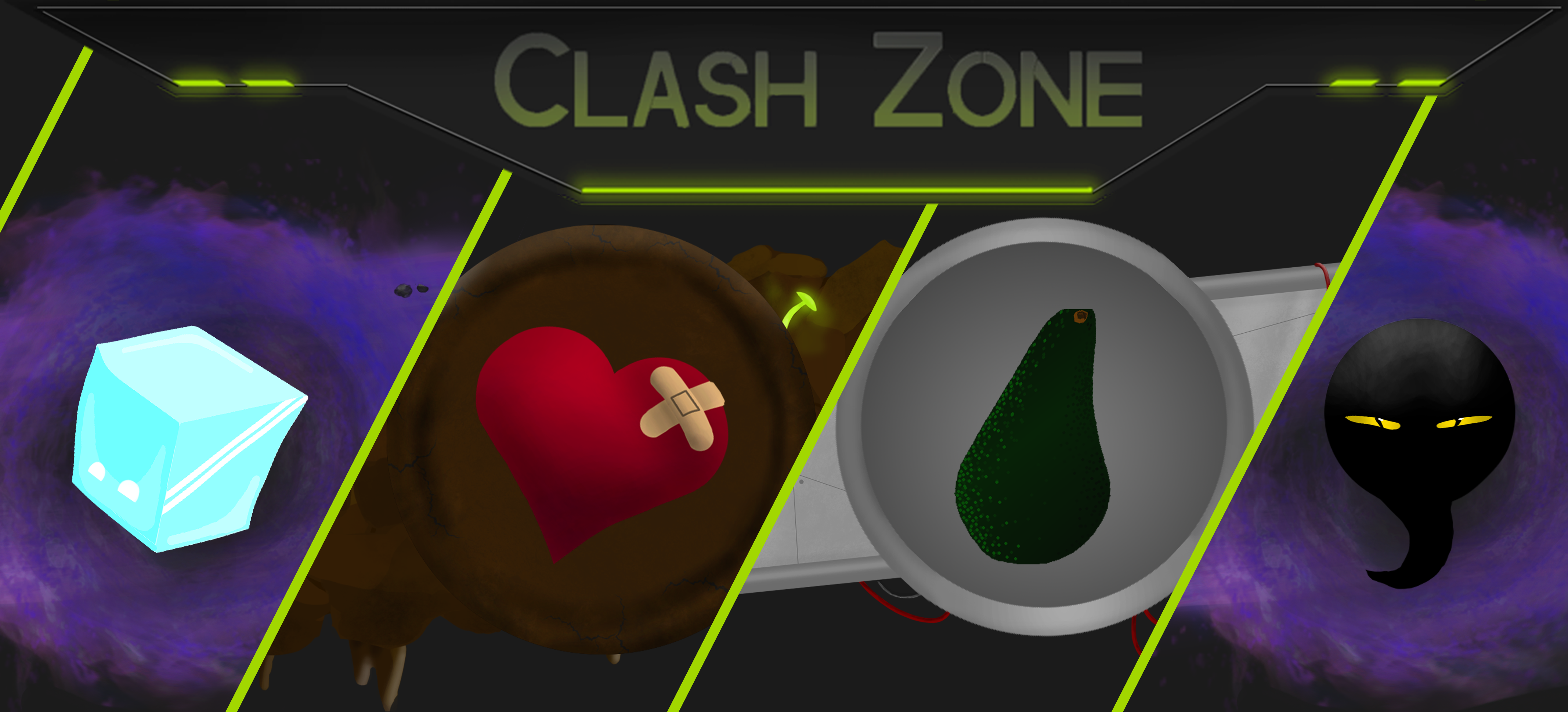The image is a digitally rendered banner likely for a game or an amusement park titled "Clash Zone" at the top. The title is in gradient gray to green lettering. Below the title, the banner is divided into four sections, each separated by bright lime green diagonal lines. 

The first section features a blue ice cube set against a purple background with a watercolor or galaxy-like appearance. The second section showcases a red heart adorned with a band-aid, placed on a brown circular backdrop. Moving to the third section, there's an illustration of a green vegetable, possibly an avocado, inside a silver circular frame with a gray background. The final section on the far right displays a circular, alien-like creature with a tail and piercing yellow eyes with black pupil slits, set against another purple background. The objects are arranged in a row, all placed upright. The entire composition has a cartoonish and vibrant aesthetic, suggesting an interactive or playful setting.